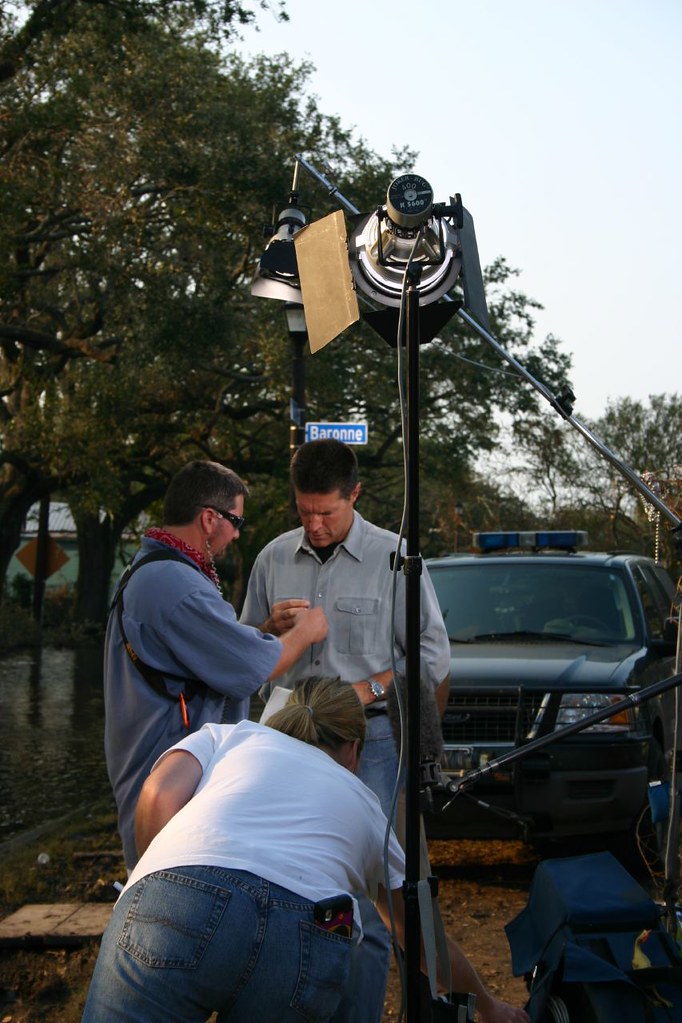The photograph appears to be taken on the set of a film or television series production in an outdoor location with natural surroundings including water and trees, possibly near a river or an area experiencing significant flooding, visible in the background on the left. In the center left of the image, a woman with her hair in a ponytail, dressed in a white t-shirt and blue jeans with a phone in her right back pocket, is bending forward facing away from the camera. She seems to be adjusting a piece of filming equipment, likely related to lighting given the tall standing light that rises above the individuals in the scene.

In front of her, two men seem engaged in a discussion or preparation. The man on the left is around 40 years old, wearing a light blue shirt with some kind of harness over his shoulders, a red paisley-pattern bandana around his neck, black sunglasses, and a wired earpiece. He appears to be handing the other man, presumed to be an actor or presenter, a microphone or another piece of gear. This second man, positioned slightly to the right, wears a pale gray button-up shirt, blue jeans, and a black belt. He has short brown hair and holds a piece of paper, seemingly reviewing notes or a script. Behind them to the right is a police SUV, identifiable by the blue lights atop, contributing to the scene's ambiance indicative of law enforcement involvement.

The bottom right of the photograph is cluttered with filming equipment, including two large studio lights positioned to enhance the lighting of the scene, suggesting a professional set-up. Despite the photograph's bustling environment, none of the individuals are looking at the camera, indicating an unposed, candid shot capturing a moment of preparation or briefing. The time of day appears to be early morning or late afternoon, inferred from the dim lighting and shadows indicating either sunrise or sunset. The overall impression is of an active and busy film set with a combination of cast and crew preparing for a scene.